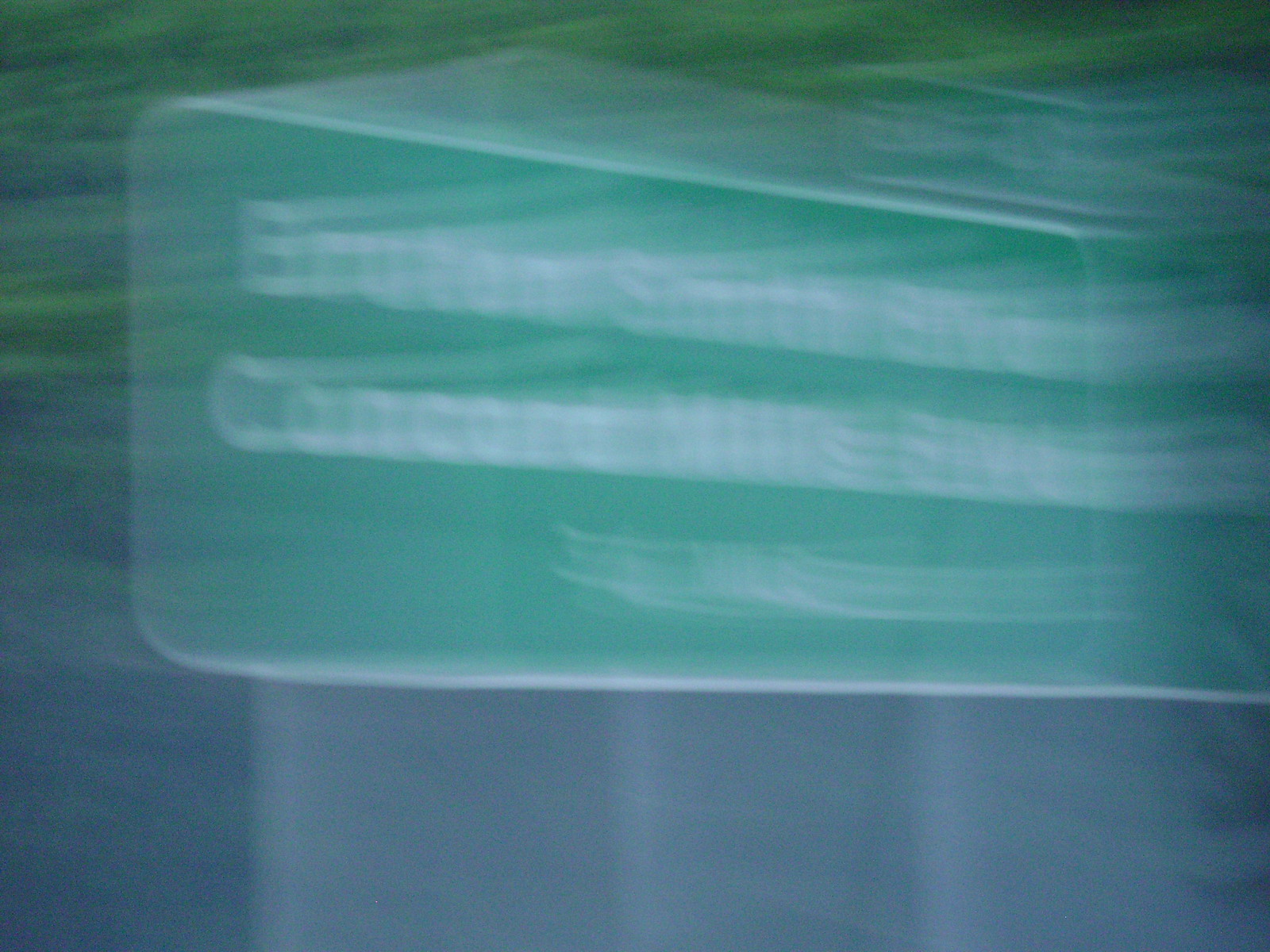This abstract artwork combines various painterly techniques and dynamic color schemes to create a thought-provoking visual experience. The lower portion of the canvas features a textured, greyish-blue area resembling the undulating folds of partially open curtains, complete with subtle lines suggesting the fabric's texture. Above this, a semi-transparent rectangle, outlined in white but filled with a rich, green hue interspersed with white lines, appears reminiscent of a translucent case or an ethereal window. Along the vertical sides of the piece, hues of green, blue, purple, and white blend harmoniously in linear patterns, adding depth and an intriguing interplay of colors. This captivating mix of textures and shades showcases the artist's skill in creating a complex yet engaging abstract composition.